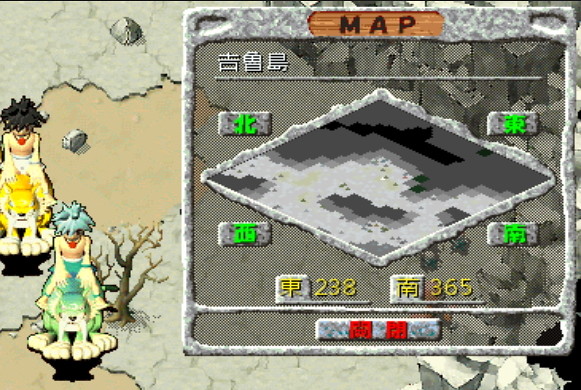This screenshot captures a scene from a simplistic video game, characterized by minimalistic graphics. In the upper right-hand corner, the word "MAP" is prominently displayed at the very top, serving as a header. Below this, the main section of the screen is largely filled with a gray background, punctuated by a distinct gray diamond shape located in the center.

In the upper left corner of the map, there are a series of characters that appear to be either Japanese or Chinese, though the exact language is uncertain. Surrounding the central diamond shape, additional characters are visible, rendered in a bright green color that stands out starkly against the gray.

Beneath these green characters, a sequence of numbers, "238" and "365," is displayed. On the left side of the screen, there are two simplistic, crudely drawn figures that resemble human beings but with notable differences: each figure has four feet, and uniquely, each foot is flat with three toes.